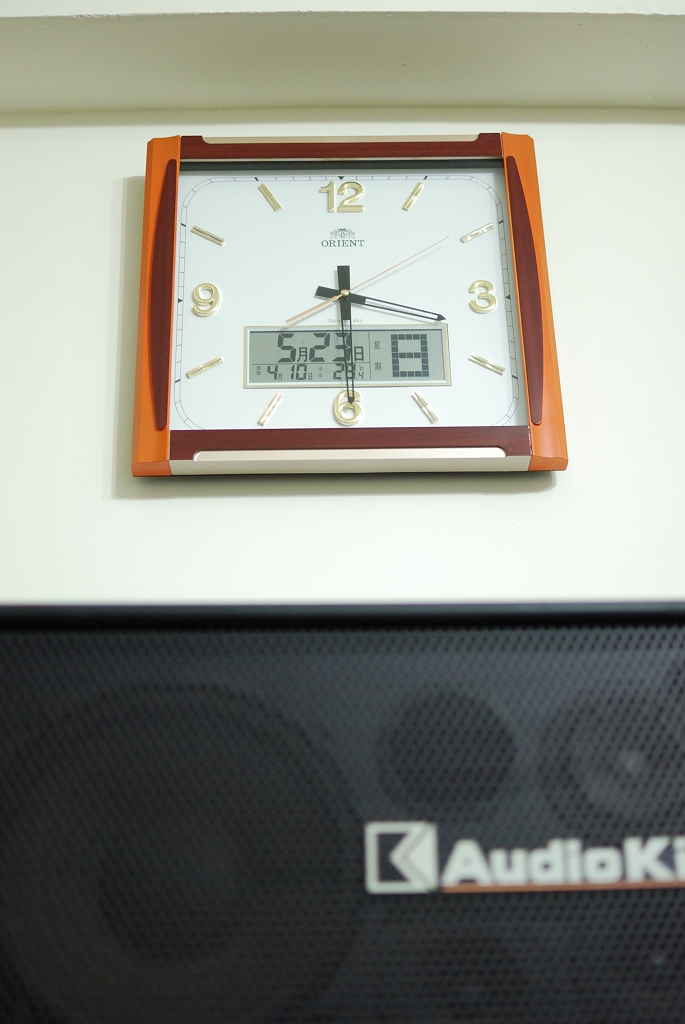The image features a sophisticated black speaker system, prominently displaying its subwoofer through a semi-transparent mesh grille. This mesh front is framed by a slightly more rigid black border at the top. A distinctive white logo, which reads "audioK" with an orange underline, is positioned on the speaker’s surface. The backdrop of the image is a pristine white wall. Mounted on this wall is a square clock with a unique design. The clock features sides made of orangish-colored wood, whereas its top and bottom edges are accented with silver. The interior wood of the clock’s frame is a darker hue. The clock face is white with gold numerals indicating three, six, nine, and twelve, while simple hash marks represent the other hours. The clock bears the brand name "Orient" in black print. Additionally, there is a digital display on the clock, which shows the current time as 5:23, along with smaller details including the date 4/10/23.